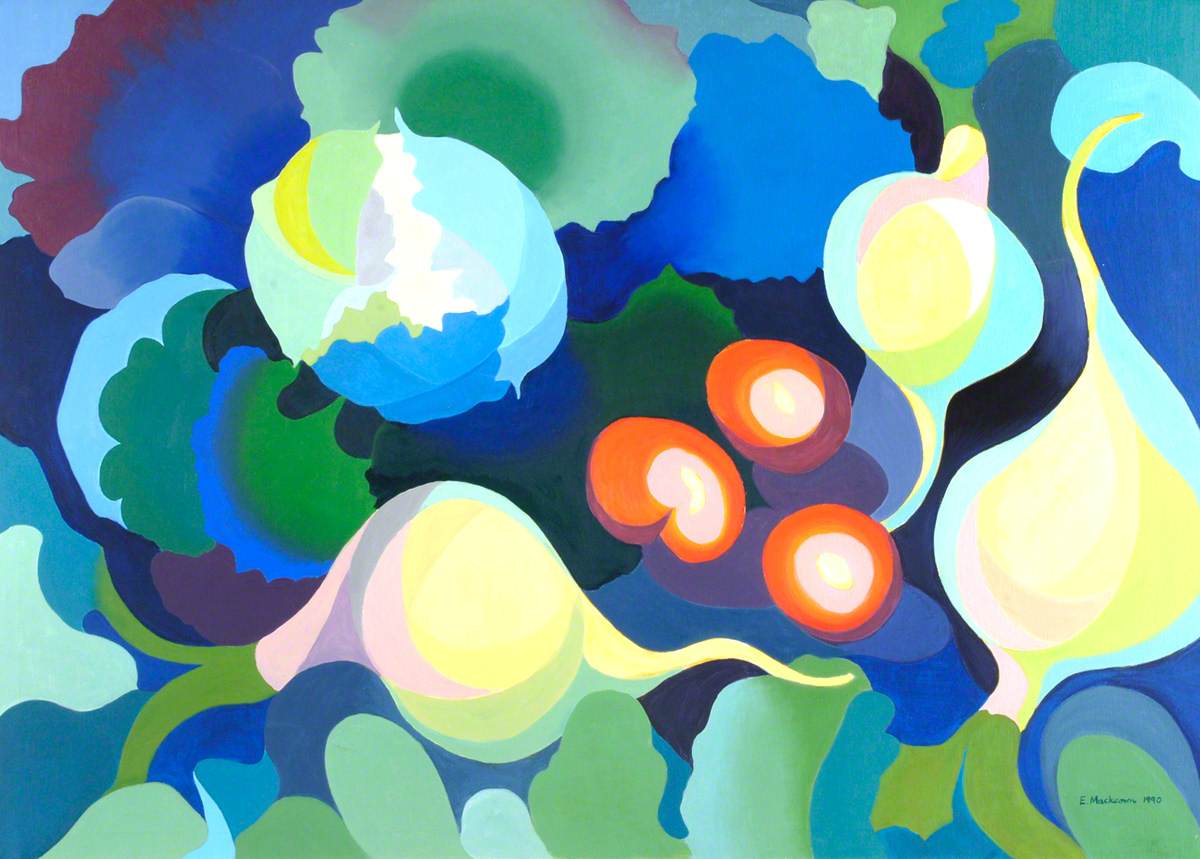The image displays an abstract painting rich in vibrant colors, featuring a variety of shapes and patterns that evoke the semblance of vegetables. Dominating the scene are several white onion-like figures sprinkled with yellow, positioned towards the middle right, bottom middle left, and also, one slightly higher and to the left of the bottom right shape. These onions appear to be sprouting, with visible green shoots emerging from their tops and green roots extending downward. Scattered around the canvas are circular forms in hues of green, yellow, orange, blue, and purple, some of which resemble Christmas ornaments or bells, and vary in size and position. Central to the composition are three round, orange shapes with pink interiors, flanking the center of the image. Additionally, a blue and white cabbage-like shape with radiating blue, light blue, and green leaves is situated to the upper left of the middle. The background is a harmonious blend of blue and green tones, enhancing the abstract, yet oddly familiar, vegetable-like forms that dominate this colorful, imaginative artwork.